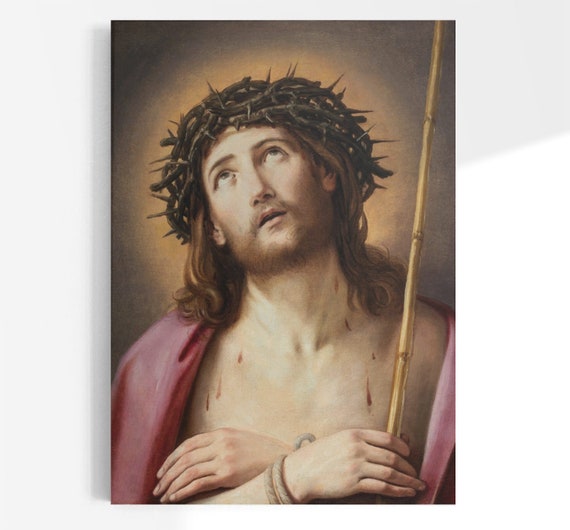This detailed, vintage oil painting in the traditional realistic style portrays Jesus Christ of Caucasian ethnicity. He is depicted with long brown hair, a beard, and a mustache, looking upwards with a serene yet sorrowful expression. A crown of thorns rests on his head, with a golden halo behind it, emitting a radiant light from his head down to his chest. His arms are bound at the wrists, overlapping over his bare chest, which is marked by droplets of blood. Jesus holds a bamboo stick in his bound hands. Draped over his shoulders is a reddish-pink cloak, standing out against the muted brown background. The profound imagery captures a moment of deep spiritual and physical suffering.